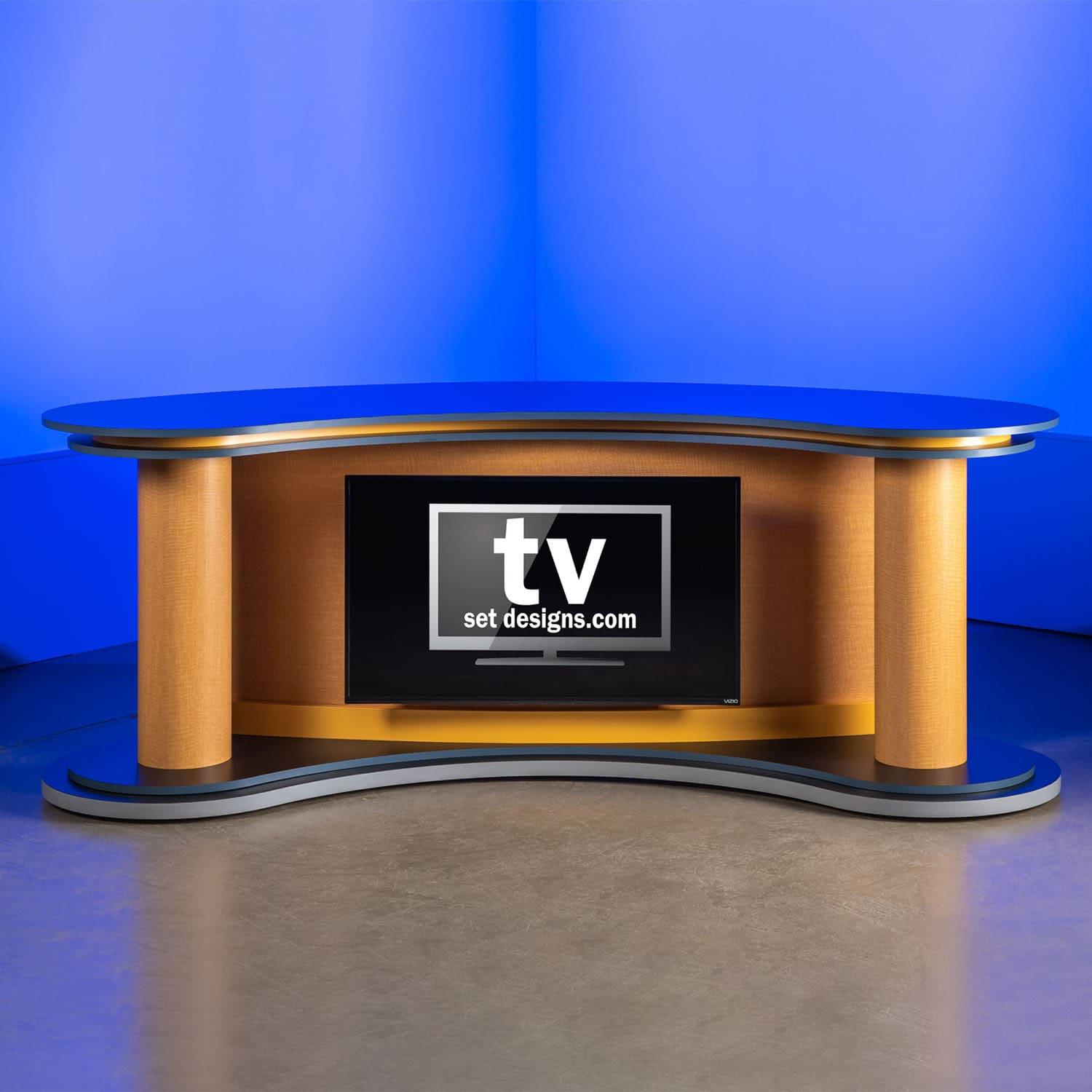The image depicts a sleek, modern TV set designed for a newscaster's desk. The set is situated in a corner of a room with polished, dark gray concrete floors. The background walls glow with a striking blue light, casting a reflective hue onto the floor and the desk. Central to the set is a U-shaped desk featuring a glass top surface and a corresponding base structure, both of which mirror the desk's curved design. The desk's base includes two cylindrical wooden columns on each side, connecting the top and bottom layers; the bottom layer is gray while the top layer is black. Located at the center of the back wooden panel of the desk is a black square, resembling a TV, which displays the text "tvsetdesigns.com" inside a drawing of a television. The top part of the desk comprises layers of black plastic and wood, enhancing its modern aesthetic. This meticulously crafted set, with its prominent glowing blue accents and reflective surfaces, is an ideal setting for newscasters to deliver broadcasts, complete with spaces for teleprompters and visual aids.